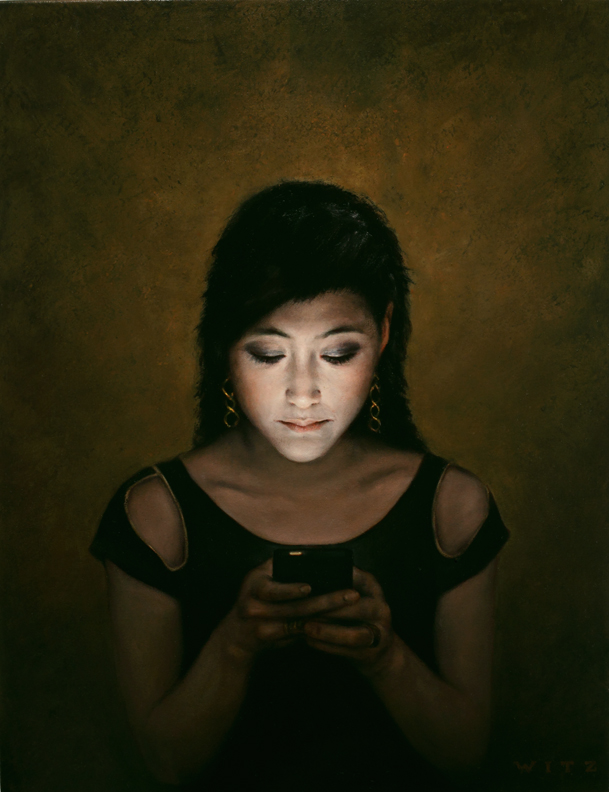In this vividly detailed and realistic painting, a teenage girl stands against a muted, bronze-brown backdrop that creates the illusion of a photographer's studio setting. The dark, shadowy environment contrasts sharply with the illumination of her face by the cell phone she holds with both hands, making her face the focal point of the composition. Her long, dark hair frames her youthful visage, adorned with dangly gold earrings that catch the gentle light. She appears engrossed in her phone, possibly texting, as she wears a sleeveless, black dress with gold trim that subtly echoes a classical style. However, the presence of the cell phone introduces a modern twist, creating an intriguing clash of eras. The dark yet elegant drapery of her dress fades seamlessly into the surrounding darkness, heightening the enigmatic and timeless quality of the portrait.